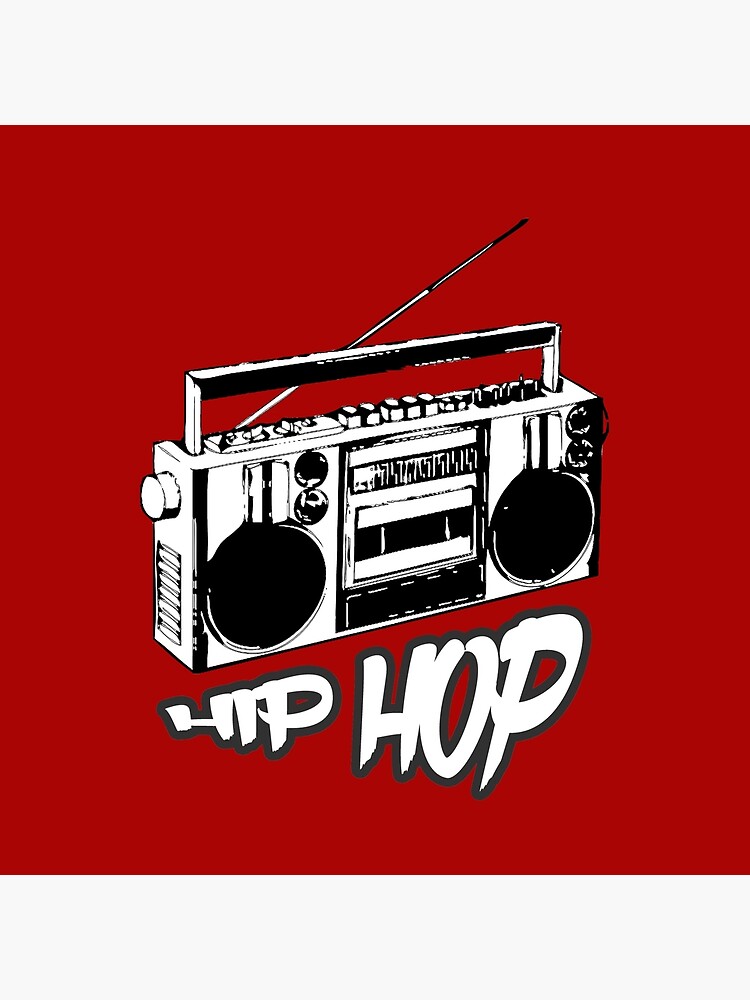This image features a detailed, black and white line drawing of a vintage 1980s boombox, prominently set against a bold red background. The boombox, illustrated in a clipart style reminiscent of cartoon graphics, showcases large black speakers on either side, a central cassette tape deck with buttons underneath, and a series of control knobs and switches at the top. A long, rectangular handle spans across the top of the boombox, accompanied by a slightly bent antenna extending upwards from the back. There is a white knob on the left side of the boombox, positioned above a rectangular grill running down the lower half. Below this detailed artwork, the word “hip hop” is boldly displayed in a unique font, outlined in black and larger at the word "hop." The entire composition is starkly rendered in black and white, set against the striking red background, creating a vivid and eye-catching effect.